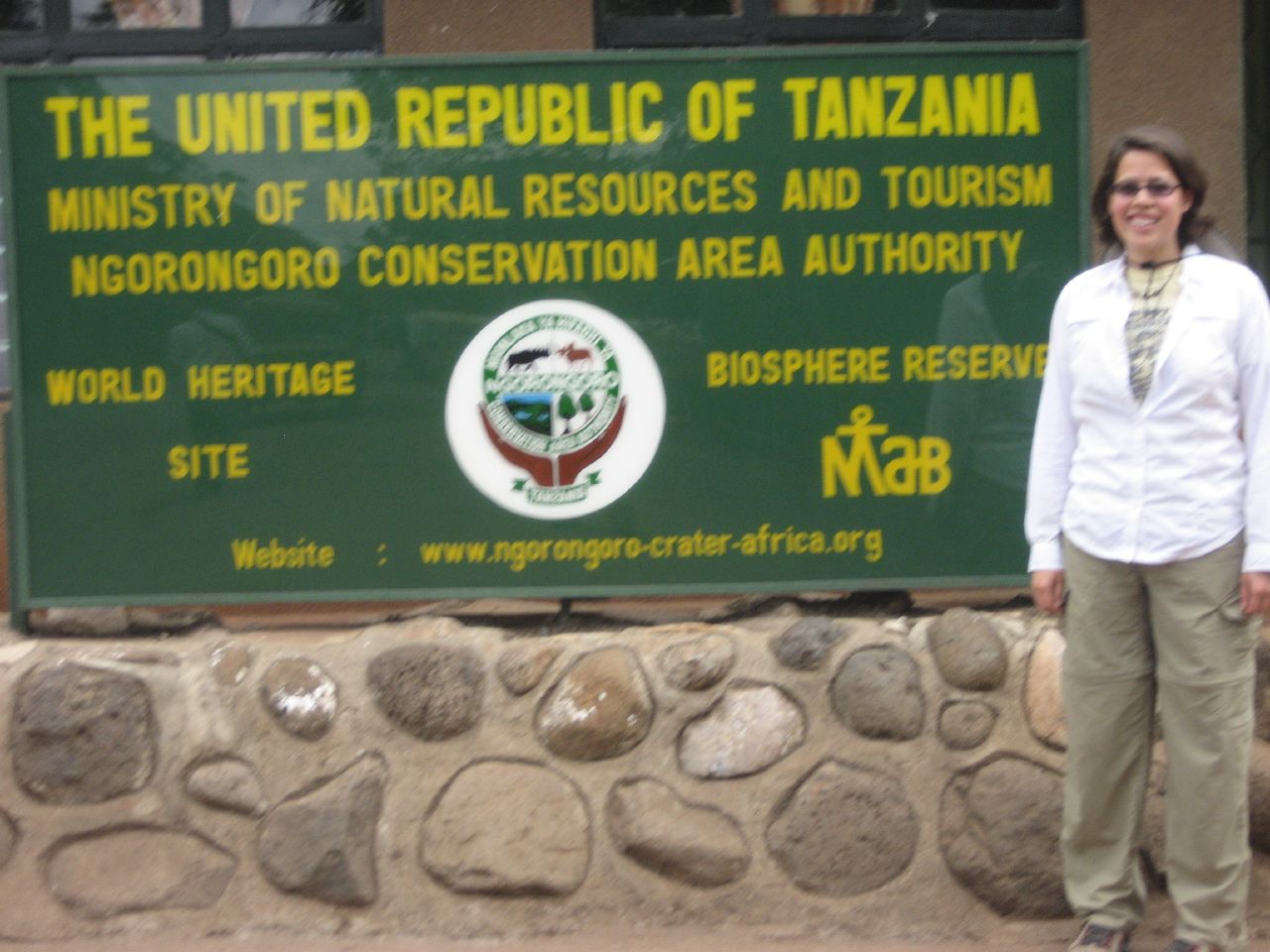In the image, a woman of medium height stands on the right, smiling broadly in front of a large green wooden sign. The sign is mounted above a stone wall that is low enough to double as a bench. The woman is dressed in a white long-sleeved shirt over a patterned shirt, paired with long khaki-colored pants and sneakers. She accessorizes with necklaces and sports short dark brown hair and tinted glasses.

The sign, adorned with yellow text, reads "The United Republic of Tanzania, Ministry of Natural Resources and Tourism, Ngorongoro Conservation Area Authority." It prominently features the place's designation as a "World Heritage Site" on the left side and notes its status as a "Biosphere Reserve" on the right. Central to the sign is a logo depicting an M where the middle leg is stylized as a human figure. Adjacent to this, another logo shows hands holding a biosphere filled with animals, plants, and water. Below these logos, the website address is displayed: www.Ngorongoro-Crater-Africa.org. The background includes glimpses of a brown building with windows, partially obscured by the sign.